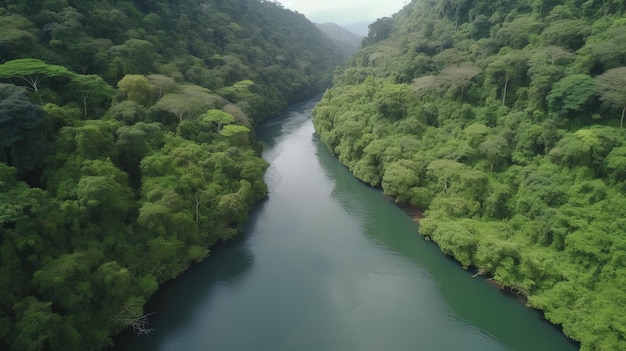The image captures an aerial view of a serene river meandering through a verdant valley, flanked by mountainous greenery. The sky in the background is a blend of gray and bluish hues, with distant silhouettes of mountain ranges against the horizon. The river, wide towards the foreground and narrowing as it stretches into the distance, reflects the sky's colors, creating an almost translucent effect illuminated by the sunlight. The water exhibits a greenish tint, contrasting starkly with the lush vegetation on both sides. The valley is dense with bright green trees and foliage, suggesting a vibrant, almost untouched natural environment with no visible buildings or human presence. The thick greenery appears diverse with trees, moss, and other plants covering the landscape, giving it a deeply overgrown and rich appearance, highlighting the pristine and tranquil nature of the scene.